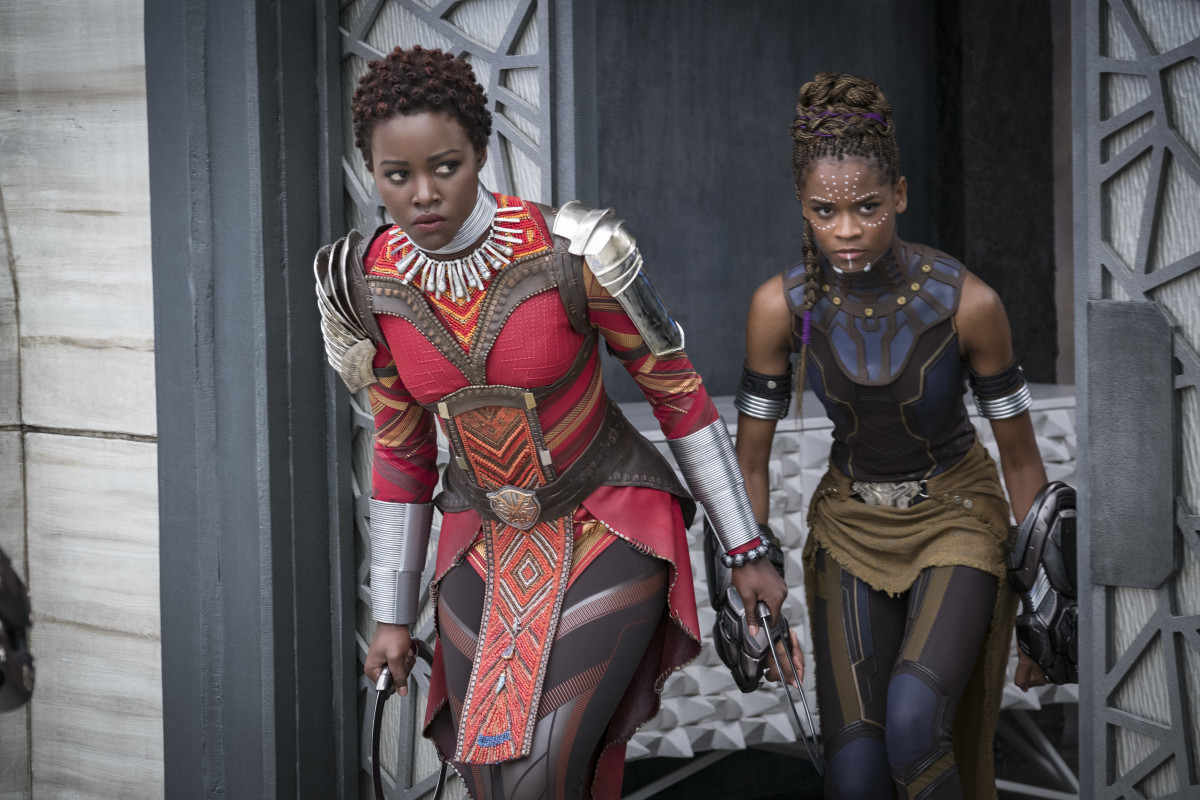In this vividly detailed still photograph from the latest Black Panther movie, we see two prominent characters, Shuri and Nakia, portrayed by actresses Letitia Wright and Lupita Nyong'o, respectively. They are depicted walking cautiously forward through a door, both in a semi-bent-over, creeping position with their eyes cast to their left—our right. Behind them, a gray doorway frames their entrance, with dark, stony textures further back. 

The actresses are adorned in striking, colorful uniforms that blend science fiction and medieval aesthetics. Shuri, on the right, is dressed in a darker outfit, with dotted white face paint and equipped with her iconic sonic gauntlets. Nakia stands to her left, wearing a vibrant red outfit, wielding her characteristic ring-shaped weapons, which resemble shields with insubstantial centers. The elaborate costumes, made of leather and latex, enhance their formidable presence, and the meticulous artistry and possible digital enhancements add to the otherworldly appearance of this potent scene.